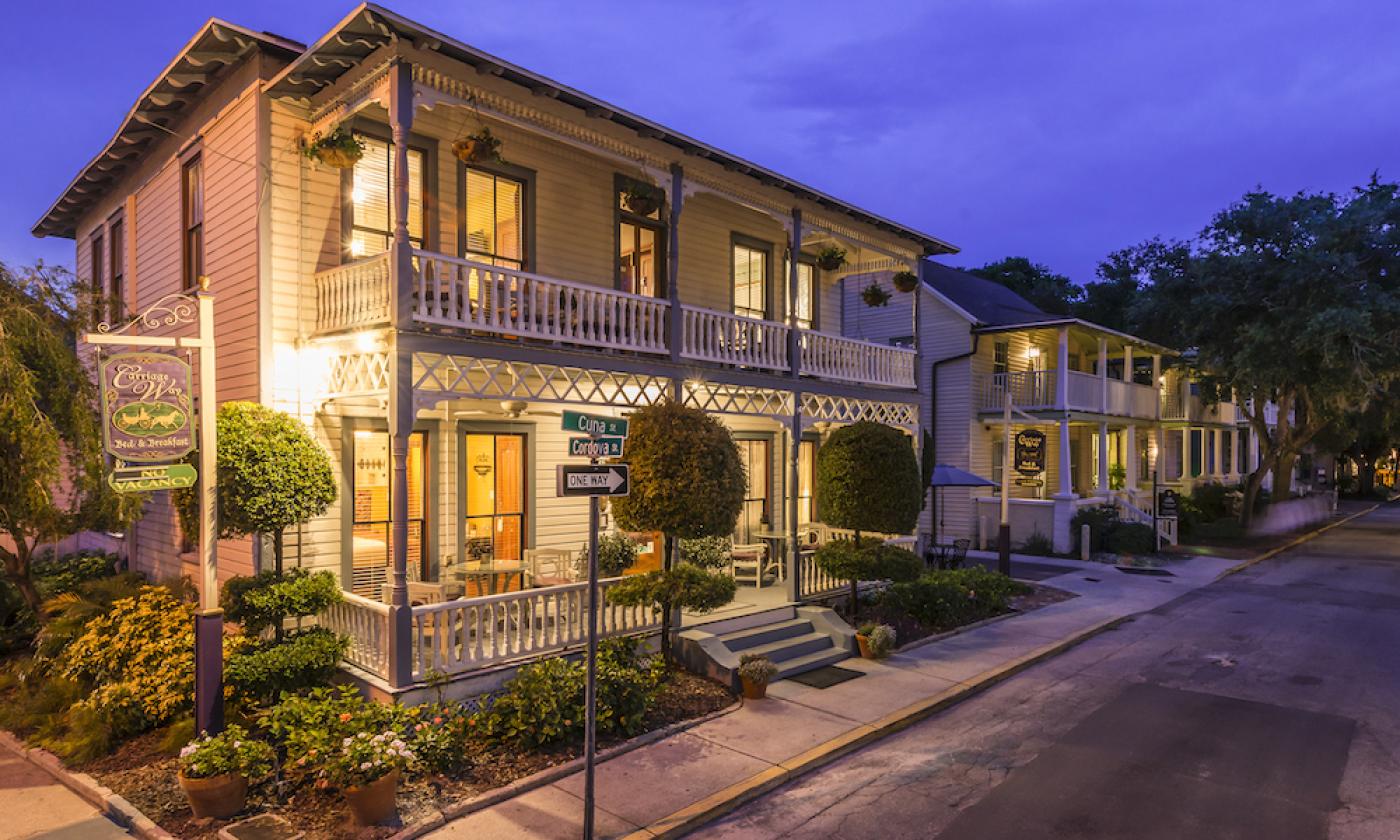This photograph captures a picturesque residential street at dusk, featuring three nearly identical American-style homes, each with a prominent double-decker porch. The house in the forefront has a rectangular shape and an inviting double decker porch, echoing a New Orleans or shore-style architecture. The sky is dark blue, hinting at the late evening setting, and the warm glow from the interior lights of the house contrasts with the dimming natural light. The front yard includes two small trees and plant beds, enhancing its inviting appearance.

The street corner is marked with signs indicating the intersection of Kuma Road and Cordova Road, and a one-way sign pointing upwards. A purple, indiscernible sign on the side of the first building, along with a "no vacancy" sign, suggests that the house might be functioning as a bed and breakfast. Further down, similar homes line the street, each with its own bed and breakfast sign, and are adorned with trees and shrubs, creating a harmonious and charming neighborhood scene.